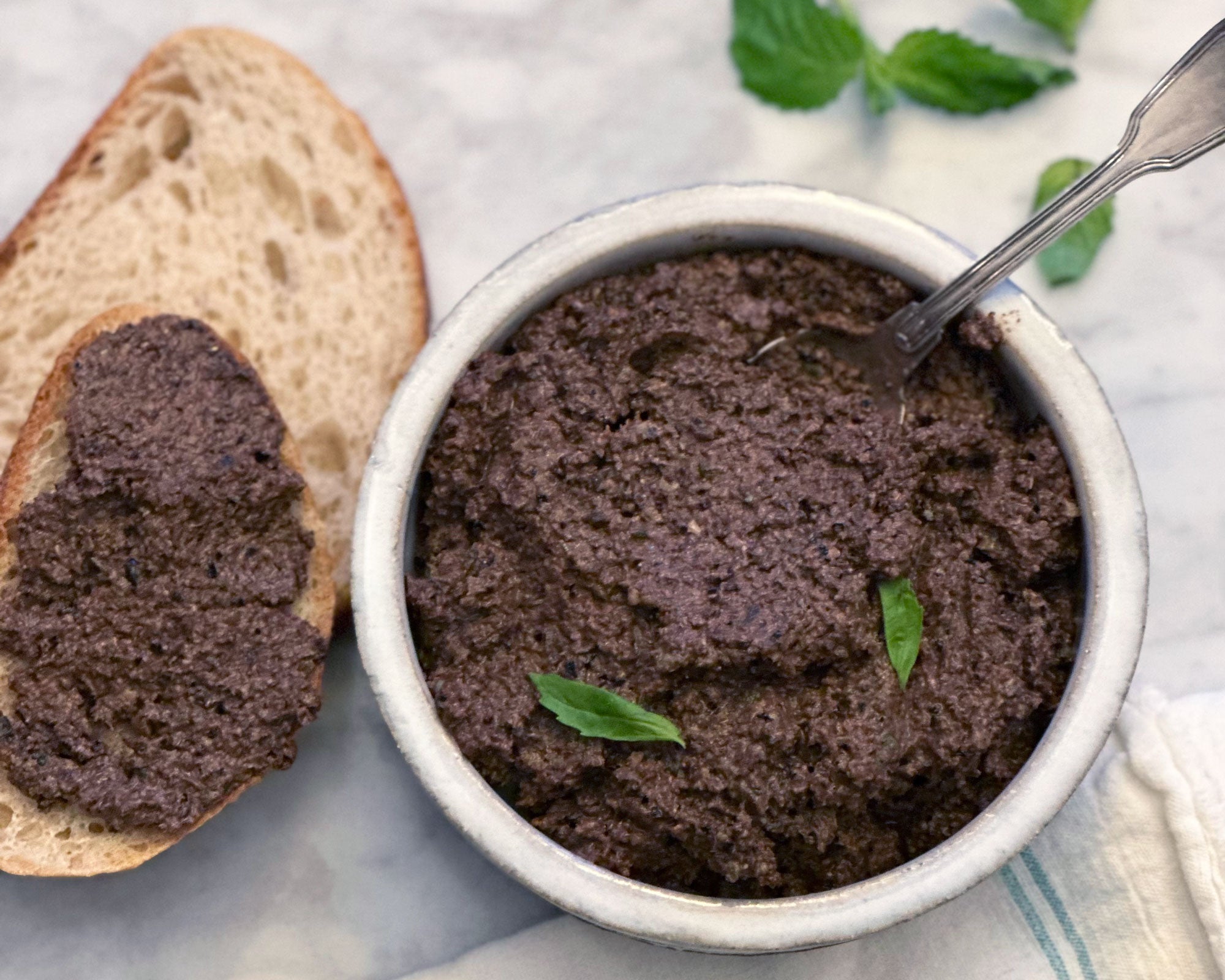The image depicts a food scene centered on a white bowl containing a dark brown spread, identified as goat cheese tapenade. This spread, which has a grainy texture, is garnished with two small green leaves likely mint. A silver spoon is partially submerged in the tapenade. Flanking the bowl to the left are two slices of baguette bread, one topped with the tapenade, the other plain, showcasing the bread's airy texture and brown crust. The arrangement rests on a white tablecloth adorned with a thin blue line, and mint leaves are scattered across the background. The table surface is white marble, adding a sophisticated backdrop to the composition.